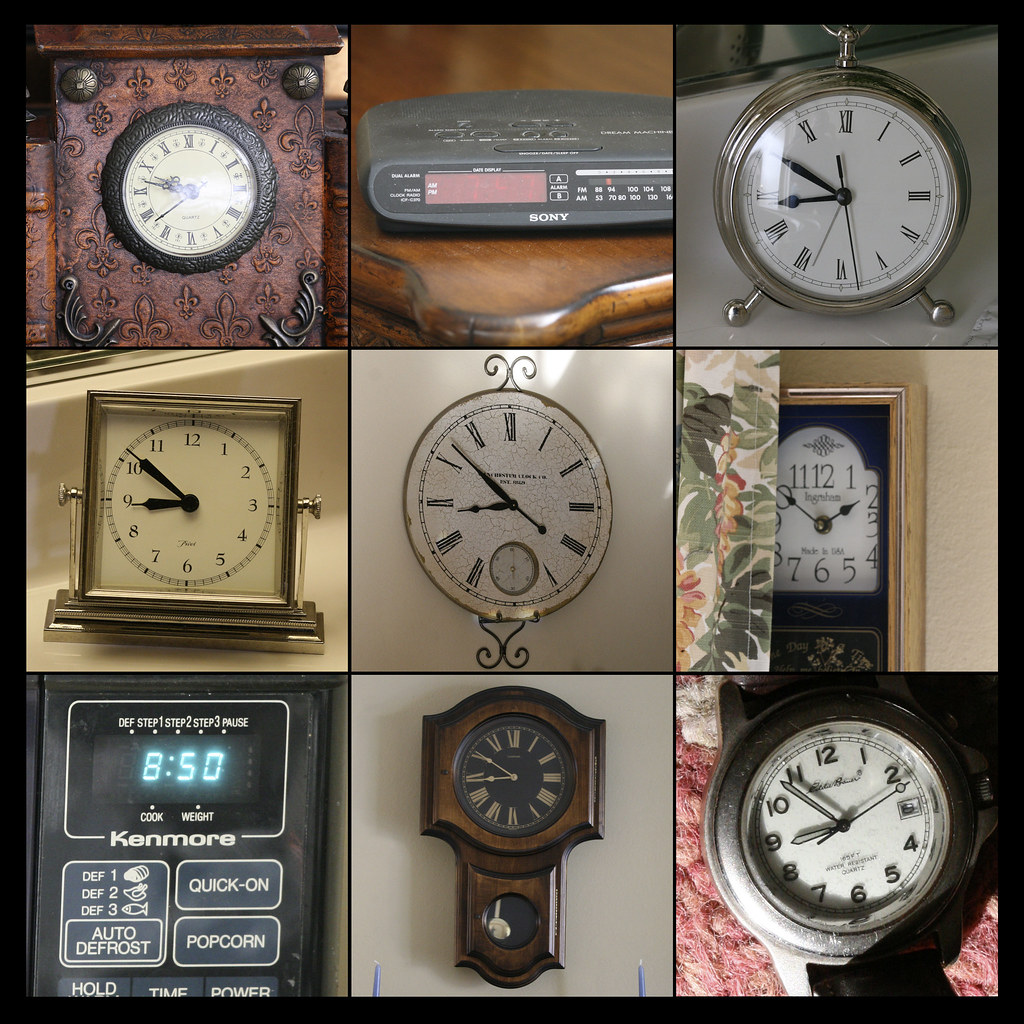This is an intricate collage featuring nine distinct clocks, arranged in a 3x3 grid, bordered in black. 

1. **Upper Left**: An ornate clock enriched with a brown wooden frame and a Fleur de Lis pattern. Its off-white face is adorned with elaborate black hands and Roman numerals from I to XII.
   
2. **Upper Middle**: A clock reminiscent of a pocket watch, silver in hue with a white face and Roman numerals. It uniquely stands on two small feet.

3. **Upper Right**: A classic pocket watch style clock in silver, characterized by a white face with Roman numerals I through XII, and also supported by two tiny feet.

4. **Middle Left**: A flat, square clock with a white face, featuring black hands, and numbering from 1 to 12 in a minimalist design.

5. **Center**: A modern digital alarm clock branded by Sony, bearing a sleek gray coloring and flat design.

6. **Middle Right**: A clock with a blonde wooden frame and a navy blue inset. It sports a traditional white face, marked with regular numbers 1 through 12.

7. **Bottom Left**: A digital readout screen displaying the time as 8:50, branded by Kenmore, resembling a microwave clock.

8. **Bottom Middle**: Two wall clocks:
   - Middle: A clock with a pure white face, Roman numerals I through XII.
   - Bottom: A wooden-framed clock with a black face, featuring a visible pendulum beneath. It also uses Roman numerals.

9. **Bottom Right**: A wristwatch showcasing a white face and regular numbers from 1 to 12, encapsulated by a brown exterior.

This diverse collection represents a range of timepieces, from ornate and classical to sleek and modern designs.